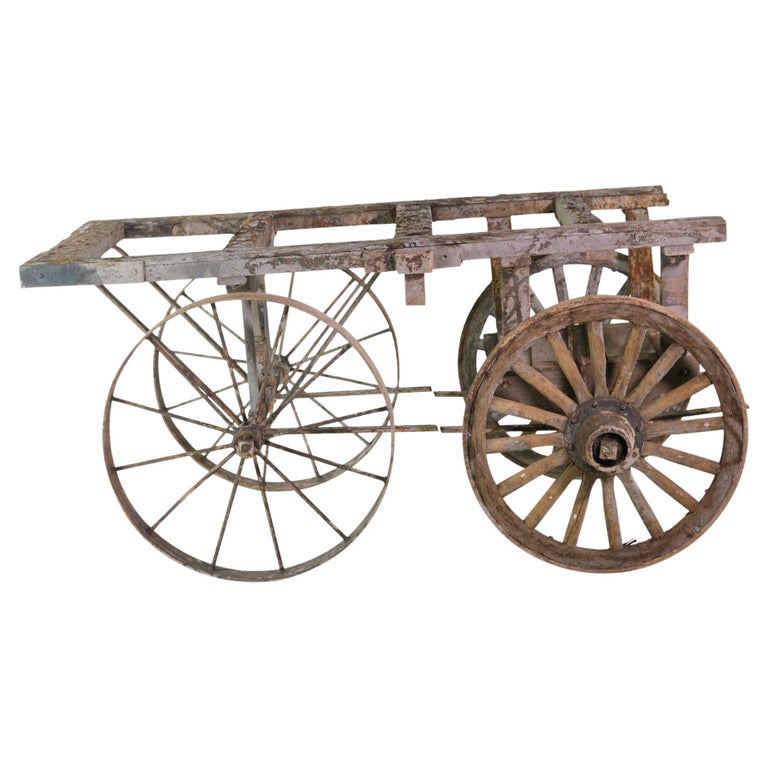This image depicts a very old, vintage cart or wagon set against a solid white background, making the subject the sole focus. The cart, appearing weathered and distressed, is constructed predominantly from wood and metal. Its frame consists of a rectangular structure with four wooden crossbeams in the middle, all displaying signs of significant wear in rusty brown and black hues. The cart features two distinctly different sets of wheels. The front (or right side) wheels are thick, solid wooden wheels characterized by a rugged brown color, with robust wooden spokes radiating from a metal hub. In contrast, the back (or left side) wheels are much thinner, made entirely of metal, and showcase a delicate design with thin spokes and a narrow metal band outlining the rim. This blend of materials emphasizes the antique nature of the cart, suggesting a piece that has seen extensive use over many years.